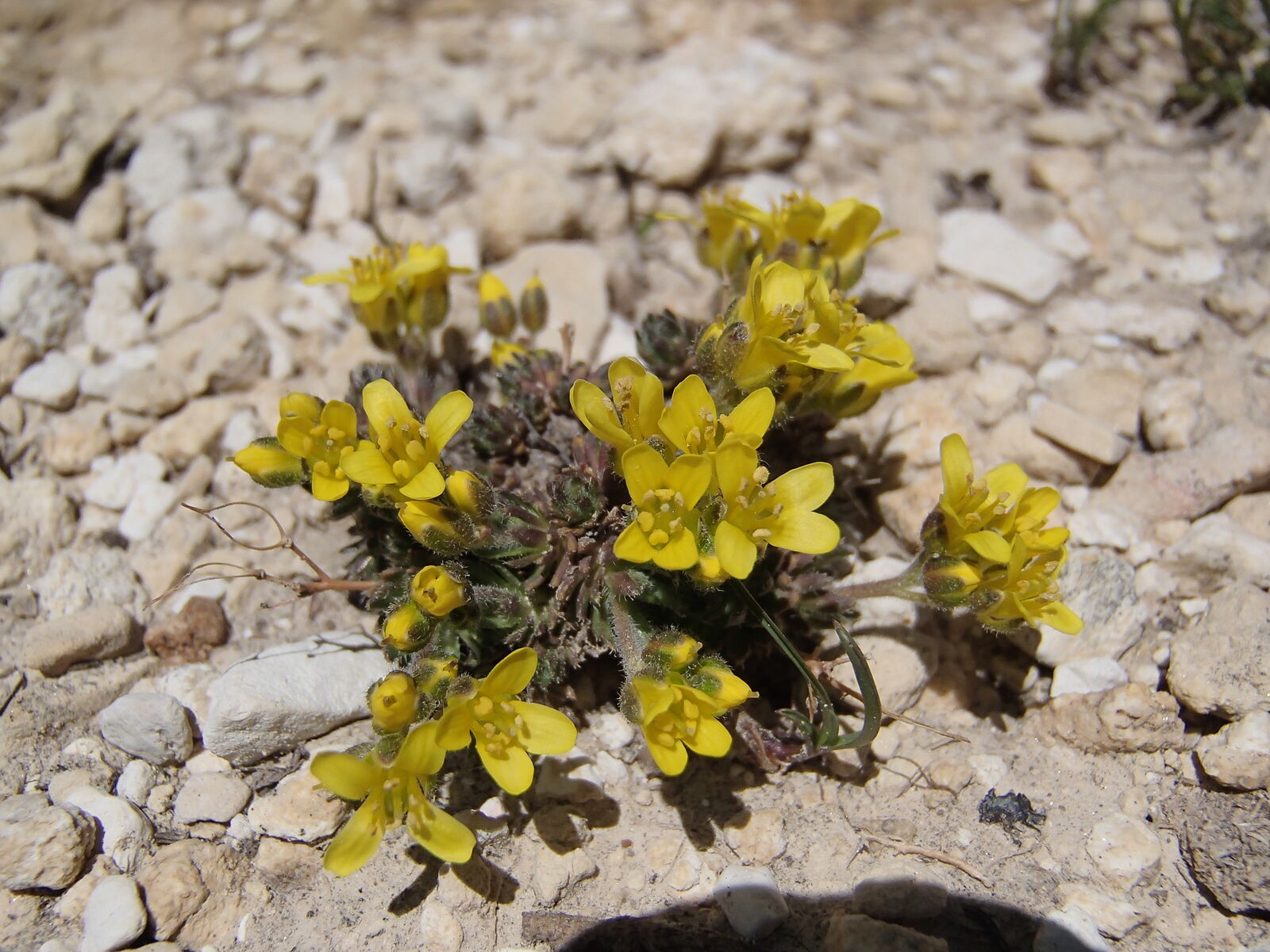The image captures a resilient little green bush emerging from a dry, rocky terrain, its stems adorned with small, vibrant yellow flowers. The ground is barely visible beneath the multitude of white, gray, brown, and tan rocks strewn around. At the bottom right corner, a curved shadow, likely from the person taking the picture, adds a human element to this top-down daytime shot. In the blurred background, more rocks of similar material fade into view, with some darker ones in the upper right corner. Despite the harsh, arid conditions, the plant's buds, both unopened and fully bloomed, stand out beautifully against the barren landscape, showcasing nature's tenacity and charm.